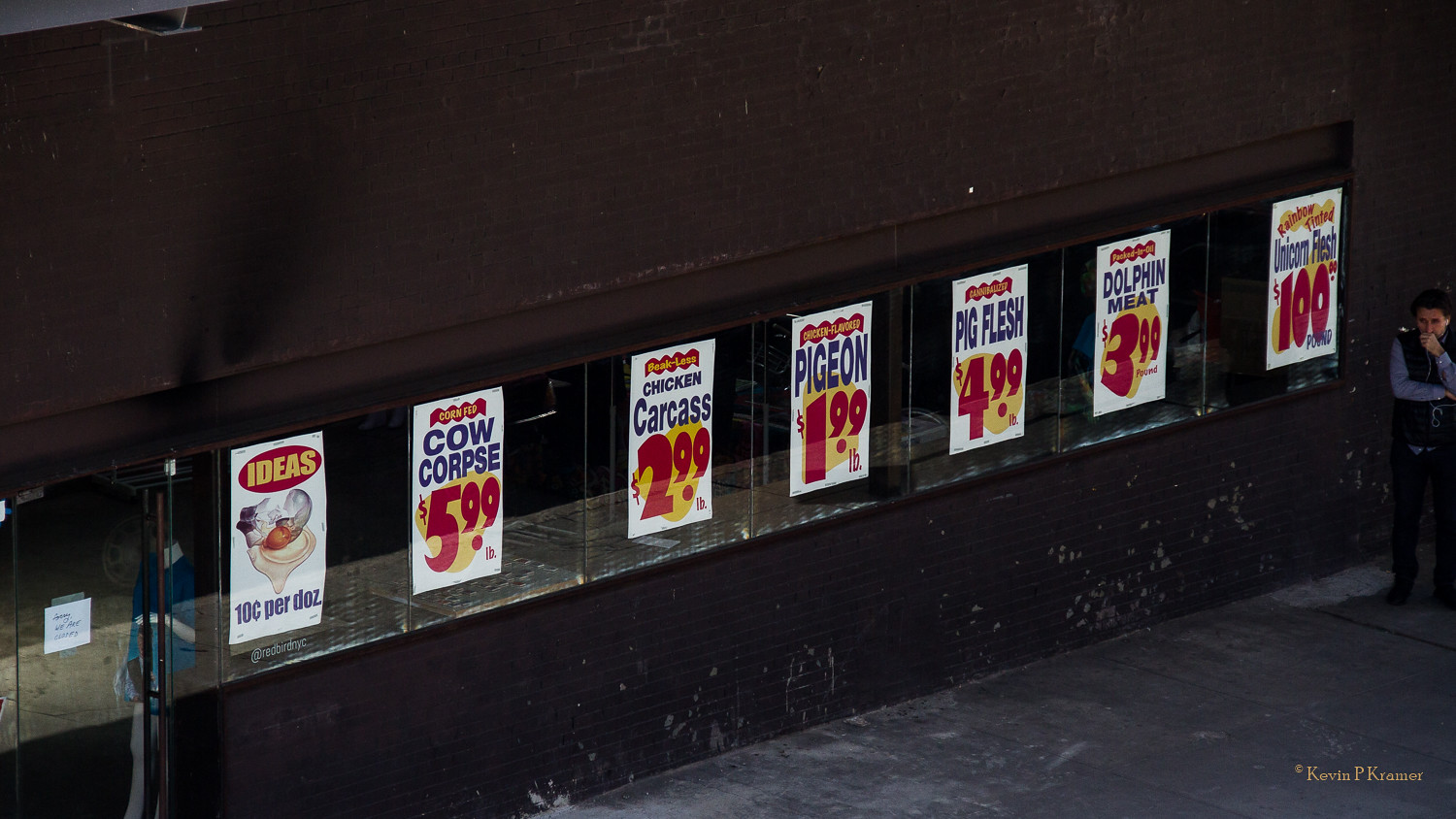This image is a digitally altered photo of an empty storefront taken from the outside. The majority of the building's exterior is covered in chipped, black paint, giving it a worn appearance. At the very top left, there is a silver or gray slit, and below it, the store features a series of glass windows and a door on the left. The windows, which have a very dark background, display several white rectangles with unusual advertisements written in blue, red, and yellow lettering. 

Starting from the lower left, the signs read: "Ideas, $10 per dozen," followed by "Cow corpse, $5.99 per pound," "Chicken carcass, $2.99 per pound," "Pigeon, $1.99 per pound," "Pig flesh, $4.99 per pound," "Dolphin meat, $3.99 per pound," and finally, "Unicorn flesh, $100 per pound." These quirky and potentially AI-generated signs add a humorous element to the otherwise bleak storefront.

On the right side of the image stands a light-skinned man with dark brown hair, dressed in a long-sleeved blue shirt, a black sleeveless zip-up vest, dark pants, and black shoes. Beside him in the bottom right corner is the text "Kevin P. Kramer" written in yellow font. This playful touch suggests the photo is intentionally absurd, blending elements of reality and fantasy.